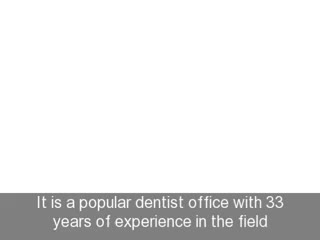The image is a predominantly white rectangular shape with a small gray horizontal text box situated towards the bottom. The white-colored text inside the box reads, "it is a popular dentist office with 33 years of experience in the field," spread across two lines. The font resembles Arial and lacks any punctuation. The background is entirely white, giving a plain, empty appearance overall, leading to the impression that this could be a screen grab from a video at an inopportune moment, capturing a frame where the visual content is not displayed.